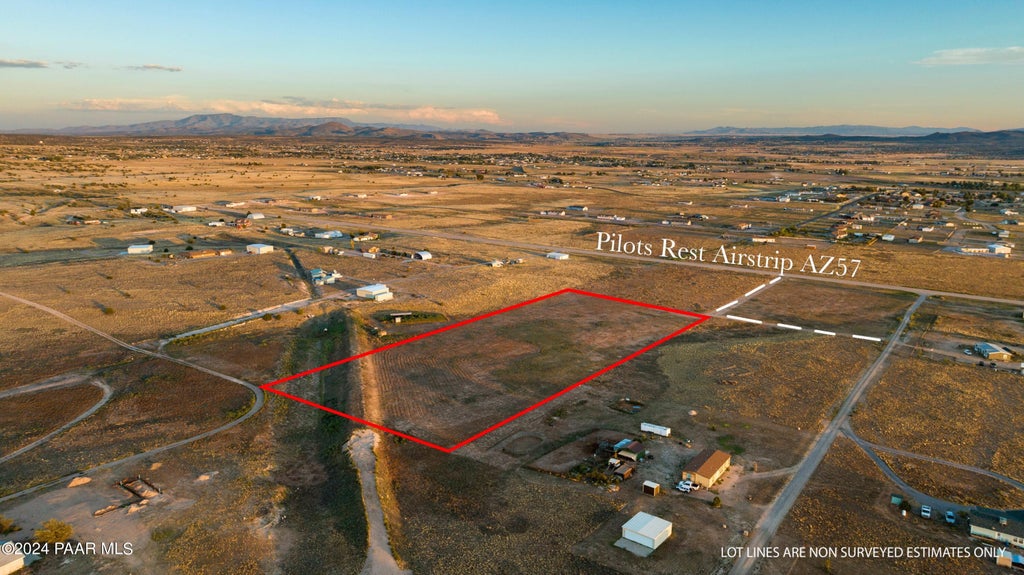The photograph is a horizontal-rectangular aerial image of a small airport, labeled "Pilots Rest Airstrip AZ-57." The ground is predominantly brown dirt, punctuated by a prominent red rectangle and various white markings, including white writing above the landing strip. The writing includes "Pilots Rest Airstrip" and "AZ-57." Scattered across the left side of the image are a few small buildings, potentially part of a very small community, surrounded by mostly barren dirt. Additionally, the image shows a few paved roads, and the buildings appear sparse and somewhat disorganized, giving the appearance of scattered debris from the aerial perspective. The top part of the image reveals a bright blue sky with some clouds near the horizon. Other details include "2024 P-A-A-R-M-L-S" mentioned in the caption, and the note about lot lines not being precise.